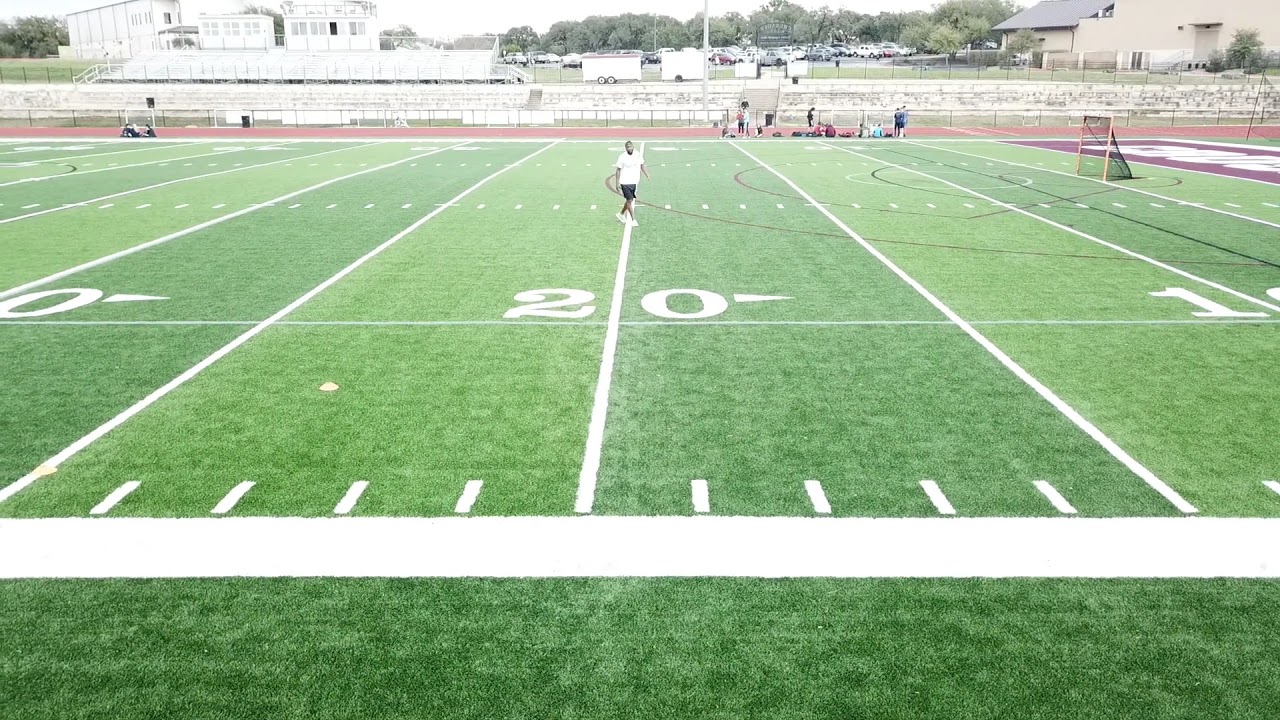In the middle of a well-kept football field made of green grass with neatly drawn white lines, a Black man wearing a short-sleeved white shirt, black shorts, and white shoes stands on the 20-yard line near the center of the field, walking towards the bottom right corner. The field features a sequence of marked lines, prominently displaying the numbers 10, 20, and 30. At the end zone, there's a soccer goal with yellow posts and a black net. Surrounding the field is an orange-colored track, and beyond it to the left, there are white bleachers and an announcer's box with multiple windows—one of which is open. Adjacent to the announcer's box is an additional building with closed windows. The upper right corner of the background showcases another cream-colored building with a brown roof, and between these structures is a parking lot filled with cars. Framing the scene further back is a line of dark green trees, under a hazy, overcast sky. The setting resembles a high school, suggesting preparations for an event or ongoing school activities.